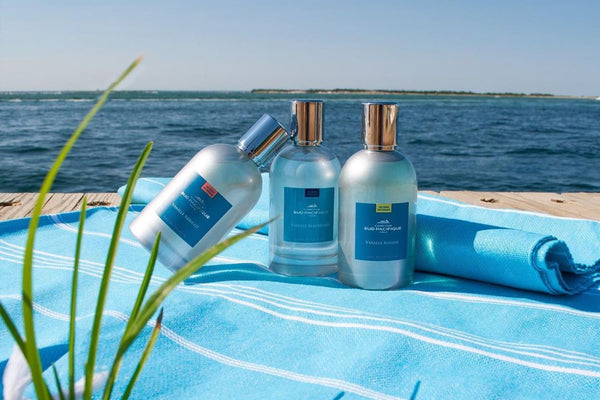An idyllic beach scene features a wooden dock extending into the ocean, framed by low, gentle waves and an island with lush greenery and sandy shores visible in the distance. The focal point on the dock is a pale blue, terrycloth beach towel adorned with white stripes, neatly spread out. Atop the towel are three bottles of health and beauty products, possibly including sunscreen, shampoo, conditioner, or body wash. Two of the bottles stand upright with one displaying a silver cap and two capped in gold, while the third bottle leans casually against the others. Though the text on the bottles is too small to read, their positioning and varied caps add to the aesthetic charm of the scene. A few strands of green grass briefly interject into the foreground, adding a touch of natural beauty to this serene and picturesque setting, which appears to be part of an advertisement.